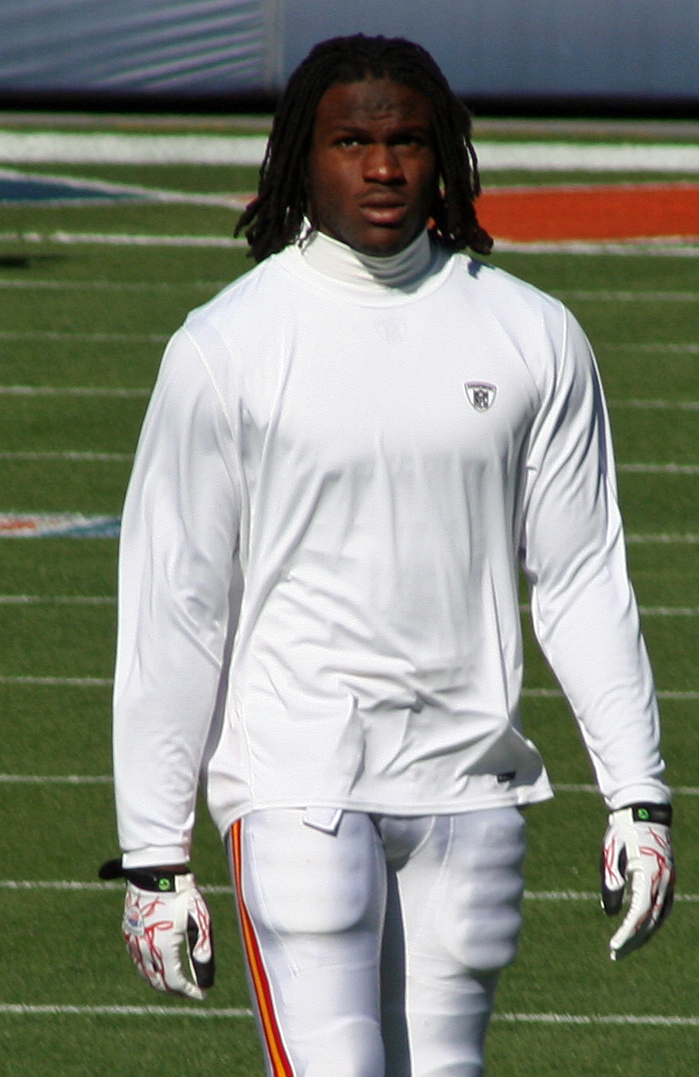In this image, a young Black man with long dreadlocks stands on a football field, wearing an all-white sporting outfit. He has a mustache and appears to be lost in thought as he looks forward, almost as if caught in a candid moment. His white long-sleeve shirt, which slightly billows as if caught by the wind, has an emblem or logo on the chest pocket that is not easily discernible. He wears padded, white football pants featuring red and yellow stripes down the sides and white gloves, likely for catching a football. The field behind him is green with white lines and includes a visible touchdown zone. In the background, there's a wall with a padded blue section and gray areas, adding to the sporting atmosphere.